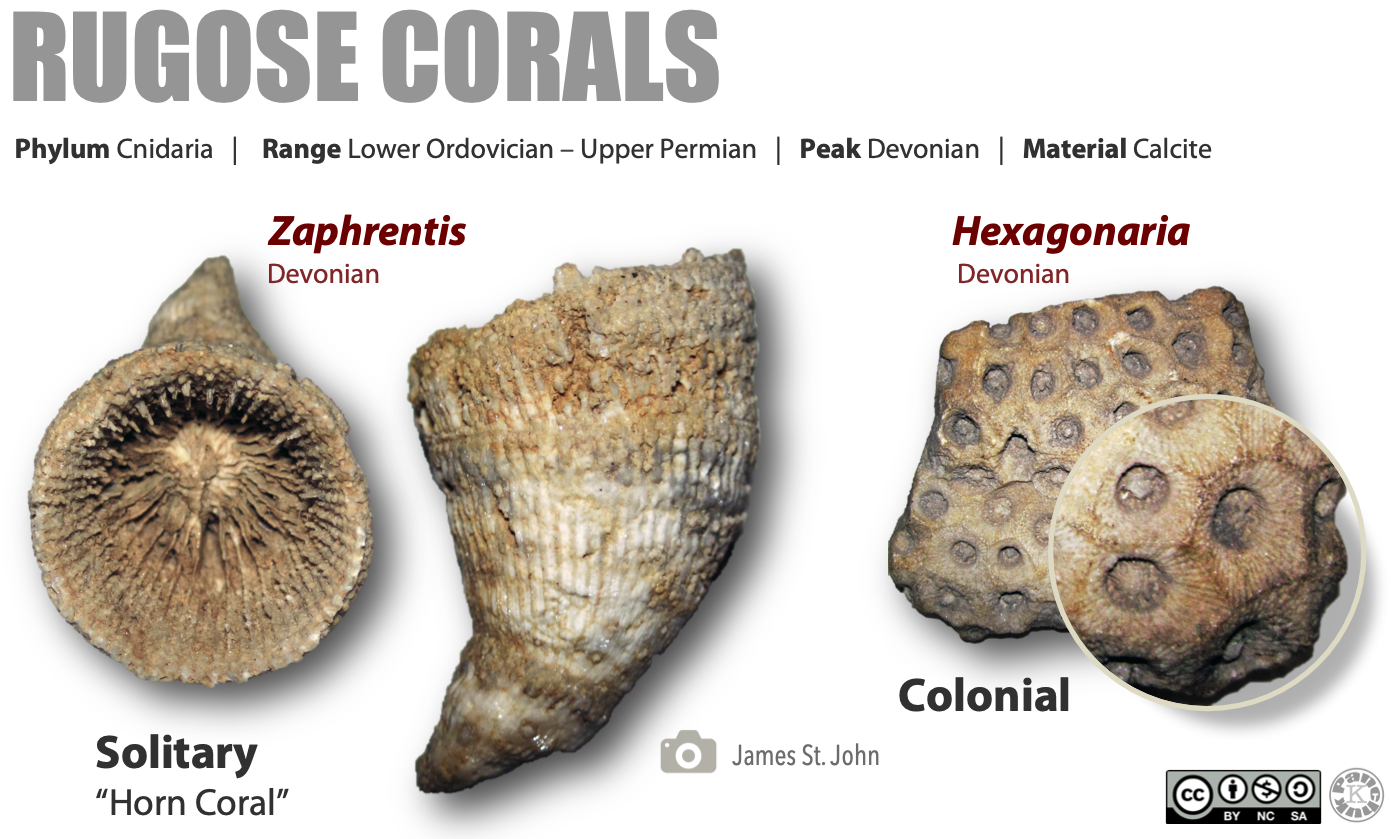The image titled "Rugose Corals" features detailed information on these ancient marine organisms. The title, in a bold gray Impact font, sits prominently at the top against a white background. Beneath it, smaller black text provides taxonomic and geological details: "Phylum Cnidaria," "Range: Lower Ordovician to Upper Permian," "Peak: Devonian," and "Material: Calcite." 

The central part of the image displays three primary types of corals. On the left and center, there are cone-shaped corals, resembling the structure of a horn, identified as Solitary Horn Coral. The scientific name provided appears to be "Zaphrentis Devonian," although it is not well understood by viewers.

Further to the right, a third coral type shows a rounded, irregular shape with a distinct black and brown dot pattern, labeled as Colonial Coral. Each of these corals has a unique texture and appearance, showcasing the diversity within Rugose corals. The image is also credited to James St. John, marked by his name and a camera silhouette at the bottom center.